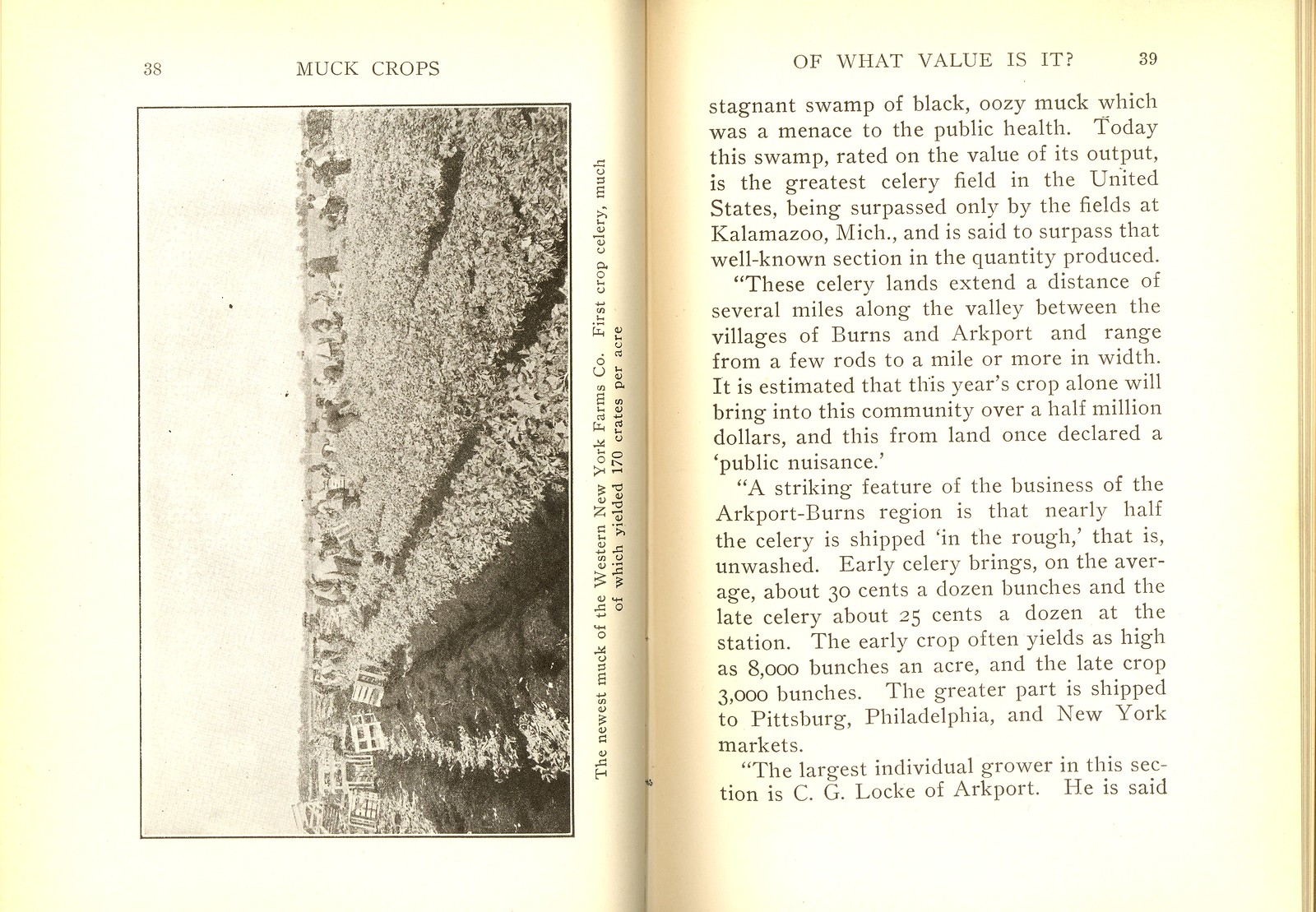The image shows an open book, displaying pages 38 and 39. On page 38, the heading reads "Muck Crops" and features a horizontally oriented photograph of farmland placed vertically on the page. This image details the newest muck land of the Western New York Farms Company with their first crop being celery, which impressively yielded 170 crates per acre. Page 39, titled "Of What Value Is It," provides an extensive text starting with "Stagnant swamp of black oozy muck, which was a menace to public health." It elaborates on the economic transformation of this once problematic land, highlighting its current status as one of the greatest celery fields in the United States, second only to Kalamazoo, Michigan. The celery lands stretch several miles along the valley between the villages of Burns and Arkport, ranging from a few rods to a mile in width, generating over half a million dollars annually from crops. The text concludes mentioning C.J. Locke of Ackport, noted as the largest individual grower in the area.